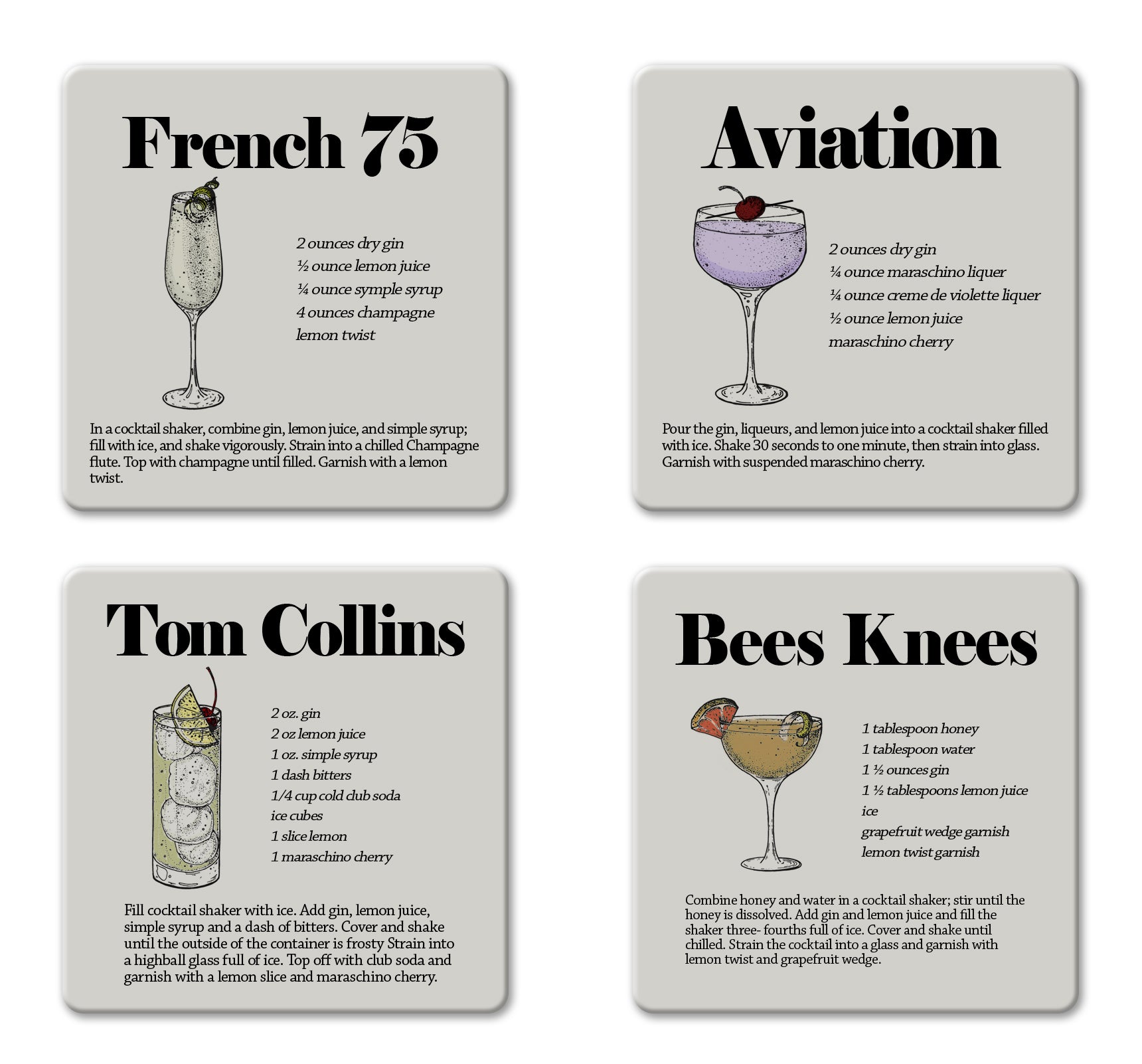The image features a set of four white coasters, each displaying an illustrated cocktail recipe. The coasters, likely the size of beer mats, are arranged on a gray background and showcase the following cocktails: French 75, Aviation, Tom Collins, and Bee's Knees. Each coaster has the cocktail name written in black text at the top. To the left of the name is a colorful illustration of the cocktail, with the colors including shades of red, purple, green, orange, and yellow. To the right of each illustration, detailed ingredients are listed, and the preparation instructions are written at the bottom of each coaster. The recipes are as follows:

1. **French 75**: A mixture of dry gin, lemon juice, simple syrup, Champagne, and a lemon twist garnish.
2. **Aviation**: Combines dry gin with maraschino liqueur, crème de violette liqueur, lemon juice, and a maraschino cherry.
3. **Tom Collins**: Made with gin, lemon juice, simple syrup, a dash of bitters, cold club soda, ice cubes, and garnished with a cherry and lemon slice.
4. **Bee's Knees**: Features a blend of honey water, gin, lemon juice, and garnished with a grapefruit wedge and a lemon twist.

The image effectively serves as an infographic, neatly and stylishly presenting the cocktail recipes with clear, concise, and visually appealing details.